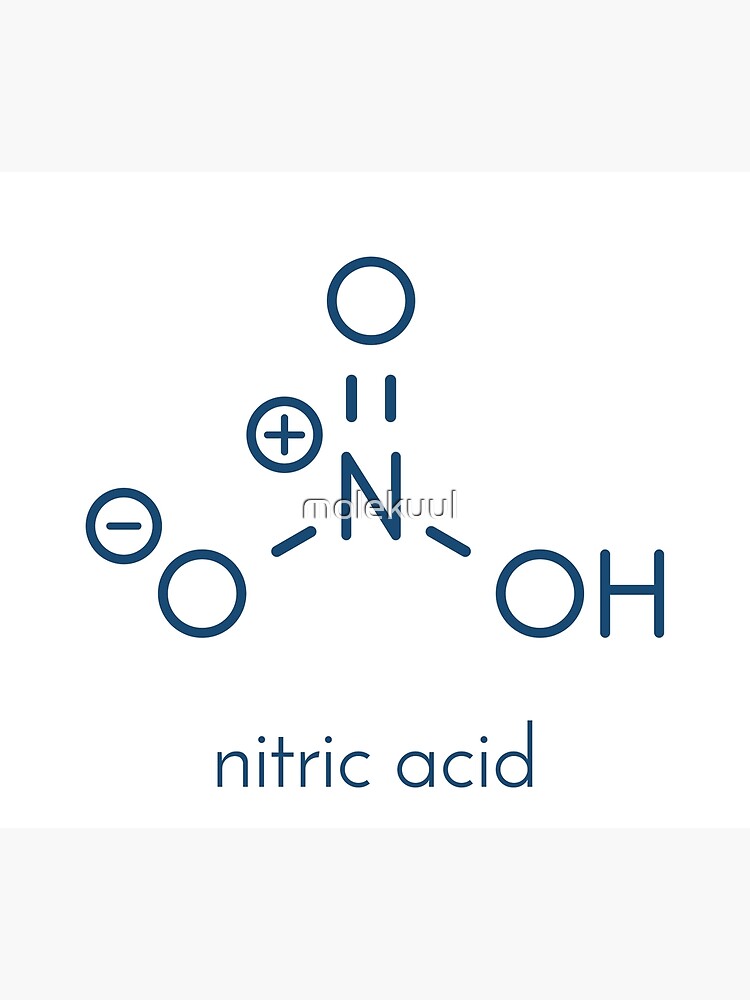The image showcases a molecular structure diagram of nitric acid against a predominantly white background, with slight grays at the top and bottom. The diagram features a prominent nitrogen (N) atom at the center, bordered by various oxygen (O) and hydrogen (H) atoms. Specifically, the nitrogen is connected to an oxygen with a plus sign and a circle to the upper left, forming a double bond with another oxygen directly above it, which has an equal sign representing a double bond. Down to the left, there's an oxygen with a negative sign in a circle, connected by a single bond. On the lower right, an oxygen and hydrogen atom are connected via a single bond. The diagram mimics the appearance of a person driving, with the plus-circled O as the steering wheel and structures resembling legs beneath the nitrogen "body." Superimposed in transparent white text across the molecular structure is the word "MOLEKUUUL." At the bottom, the caption "nitric acid" is displayed in blue text.